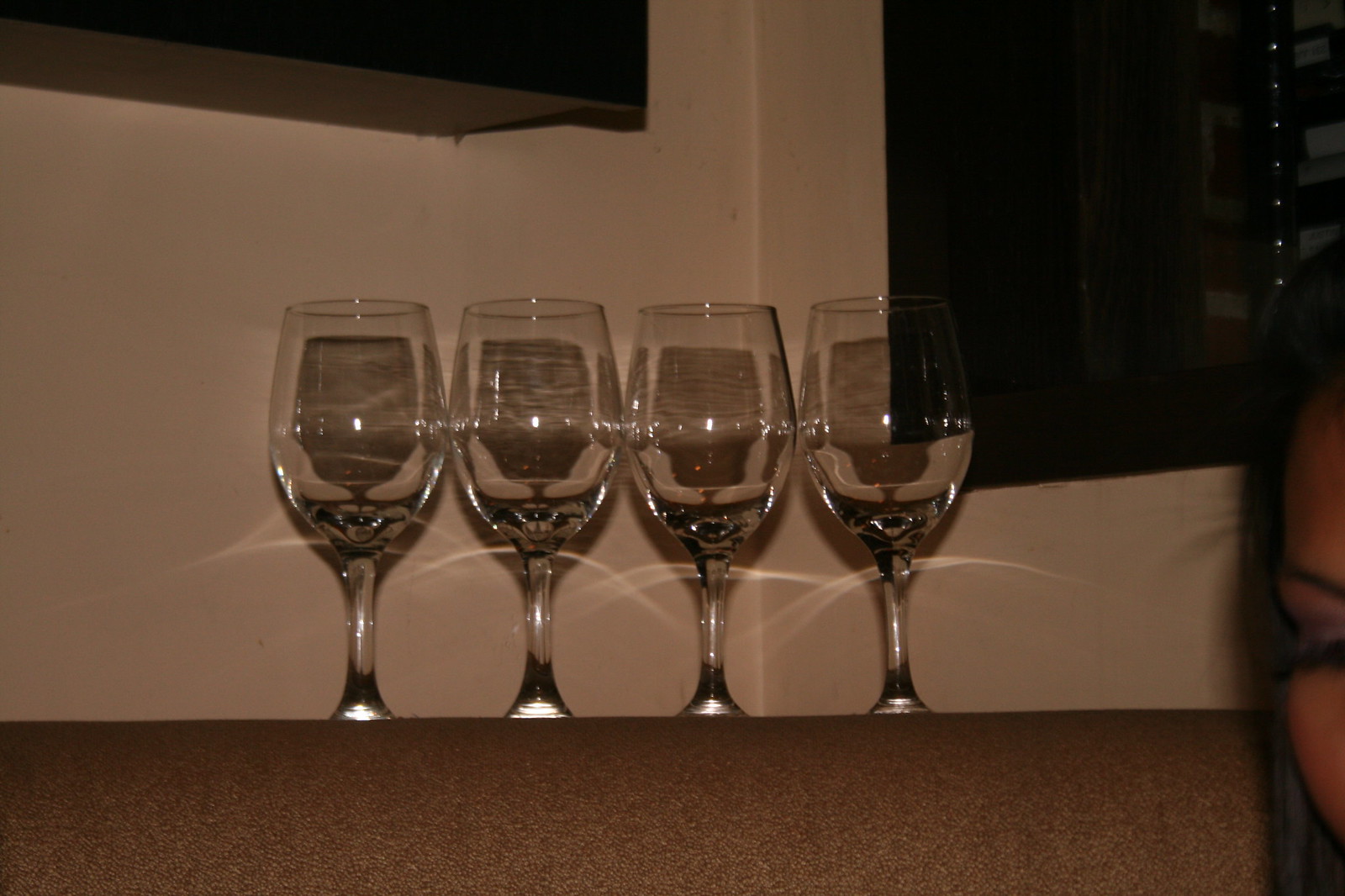This color photograph, taken inside a dimly-lit building, likely a restaurant or similar setting, features four clear wine glasses arranged in a row on a brown shelf. The shelf, possibly wooden or covered with fabric, stands out against the background, reflecting ambient light that creates delicate shadows and arc reflections beneath the glass stems. The glasses are positioned in front of a white wall with black trim, adding contrast to the scene. In the far right corner of the image, a woman with long dark hair partially obscures the background, her face angled toward the camera with her eyes closed. A piece of wooden furniture and an unlit TV can be seen behind her. The overall composition is centered on the wine glasses, capturing their clarity and the subtle interplay of light and shadow.